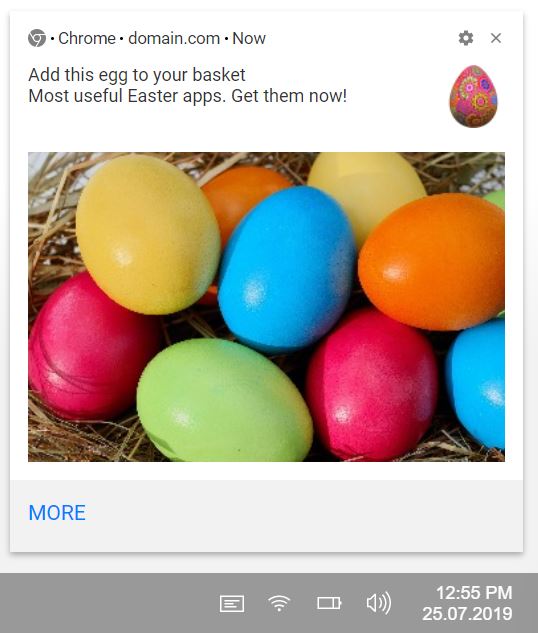**Detailed Caption:**

This appears to be a screenshot taken from a mobile phone displaying a promotional Easter-themed webpage. The top section of the screenshot includes a gray-colored version of the Chrome browser icon followed by a dot, then the word "Chrome," another dot, the text "domain.com," and another dot separating this from the text "NOW," all in uppercase with 'NOW' also capitalized. To the right of this text string are two icons: one depicting settings and another representing an 'X' which provides an option to close the view.

The content beneath this header is a promotional message written in a gray font on a white background. The message reads: "Add this egg to your Easter basket," followed by another line urging, "Most useful Easter apps. Get them now." Below this message is an image of a multicolored Easter egg with intricate designs.

Further down, there is a decorative image displaying a collection of shiny, brightly colored Easter eggs arranged on what appears to be a bed of Lexington straw. The image shows two pink eggs, two yellow eggs, two orange eggs, two blue eggs, and a single green egg.

Below this image is a banner with the word "MORE" in all capital letters highlighted in blue color. At the very bottom of the screen, the phone's status bar is visible, showing a battery life at approximately two-thirds capacity, sound turned on, and the date and time as 2:55 p.m. on July 25, 2019.